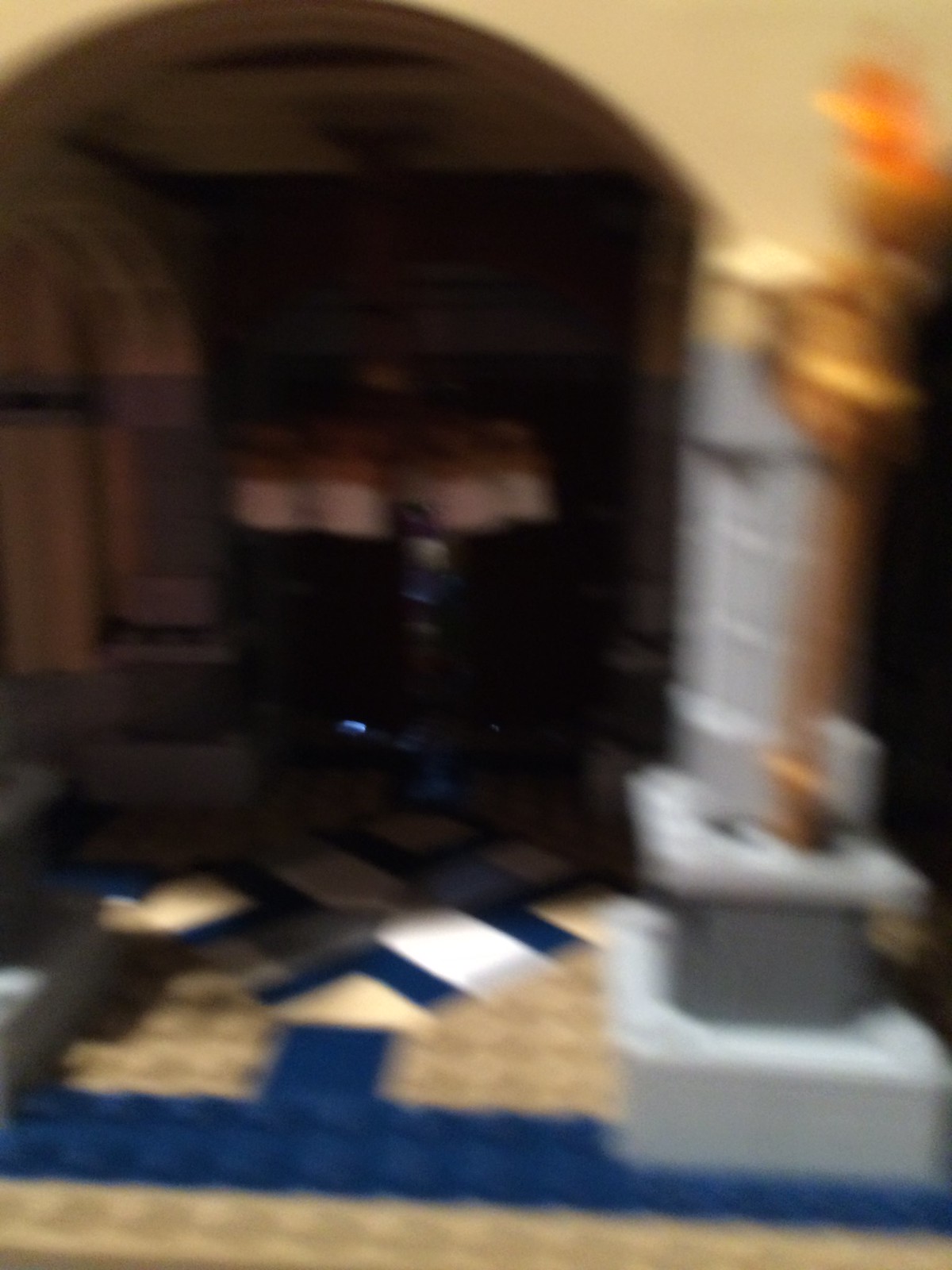In this slightly blurred color photograph, we see a partially constructed Lego set on a surface. The base of the structure is made up of tan tiles. A striking blue section runs horizontally through the center of the scene, providing a visual anchor. On the right side, gray columns rise up, adding an architectural element. Just above, a brown sphere appears to ascend, drawing the eye upwards. Amidst the assembly, the blurry shape of a flame in golden orange hues gives a sense of dynamic movement. In the background, a brown stucco archway frames the scene. Through this archway, a gray and tan statue fashioned from multiple Lego blocks is visible, with additional dark brown blocks complementing the color palette. The interplay of these elements creates a visually compelling and rich composition.